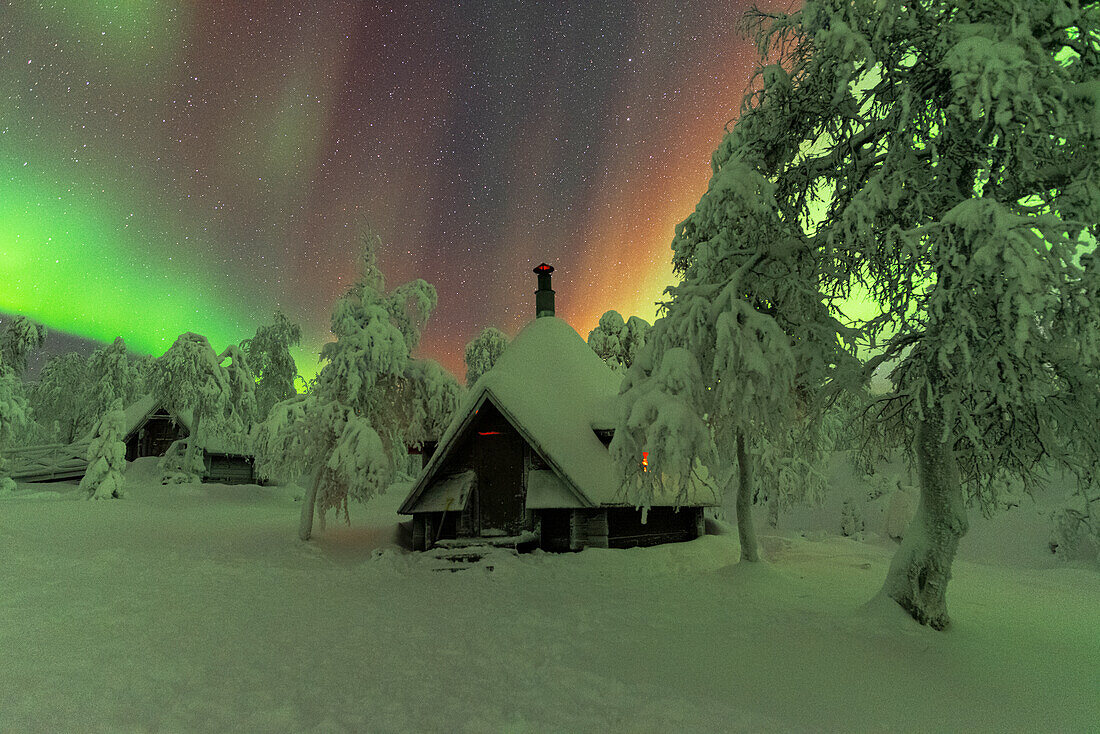This stunning photograph, possibly taken near the North or South Pole, features a breathtaking display of the aurora borealis illuminating a star-filled sky. The captivating night sky transitions through a spectrum of colors—pale green, gray, purple, peach, and various hues of green—overlapping with countless twinkling stars, suggesting a magical, unedited spectacle. In the foreground, a serene, snow-cloaked landscape unfolds. Evergreen trees, enveloped in thick layers of snow and frost, stand on either side, their branches indistinguishable under the icy covering. Nestled amidst this wintry scene are quaint cabins. The centerpiece is an adorable alpine house with an extremely peaked roof, fronted by inviting steps leading to a warmly lit front door and windows. To the right, another cabin, shrouded in snow, remains unlit. The whole scene is bathed in the soft, mystical glow of the auroras, creating an irresistible, enchanting atmosphere perfect for a cozy winter retreat.